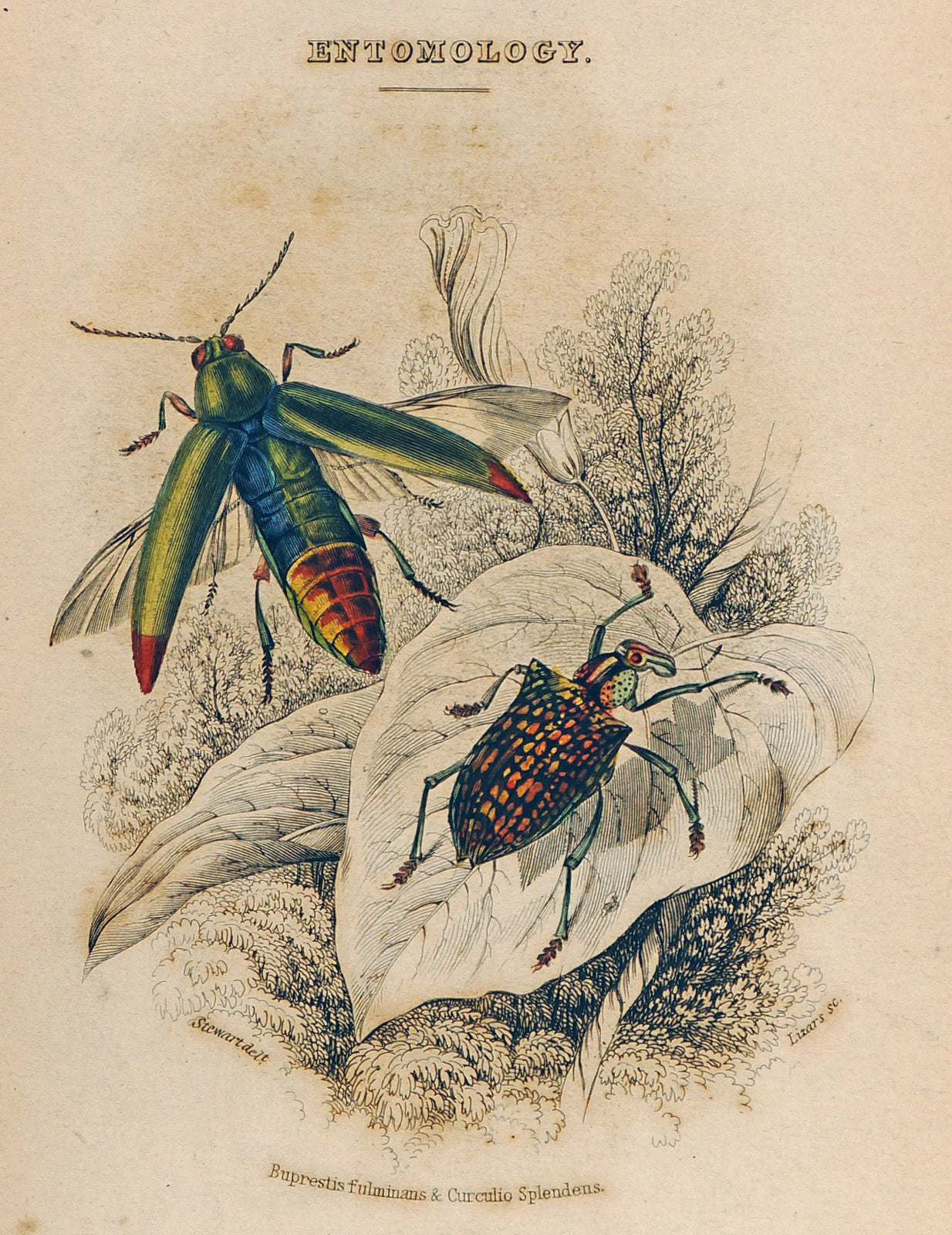The image features a detailed, color illustration on a light tan background that gives an impression of aged, browning paper. At the top, in black outlined letters, it reads "Entomology," while the bottom showcases the scientific names "Buprestes fulminens" and "Curculio splendens" in a distinctive, curved brownish text. In the foreground, there are two prominently depicted insects.

The first bug, resembling a stink bug with a shield-shaped body, is perched on a large, eye-catching leaf. Its black body is adorned with yellow and orange dots, and its head stands out with white markings accented by black and orange. This insect is wingless and features legs with hook-like structures for gripping the leaf.

The second insect is suspended in mid-air nearby. It has an elongated body with vibrant blue, green, and yellow coloration. Its thorax is segmented with striking orange and black colors, while its wings are vivid green with red tips, and it also possesses clear wings rimmed with black. The head of this bug is green, marked by piercing red eyes, and it has prominent pincers.

In the background, a large tree and various plants, including the giant leaf with the perched beetle, add to the authenticity and intricate detail of this entomological illustration. Notably, in the left-hand corner, the name "Stuart Dell" appears, with "Lizards SC" inscribed on the right, adding a touch of personal or artistic attribution to the image.